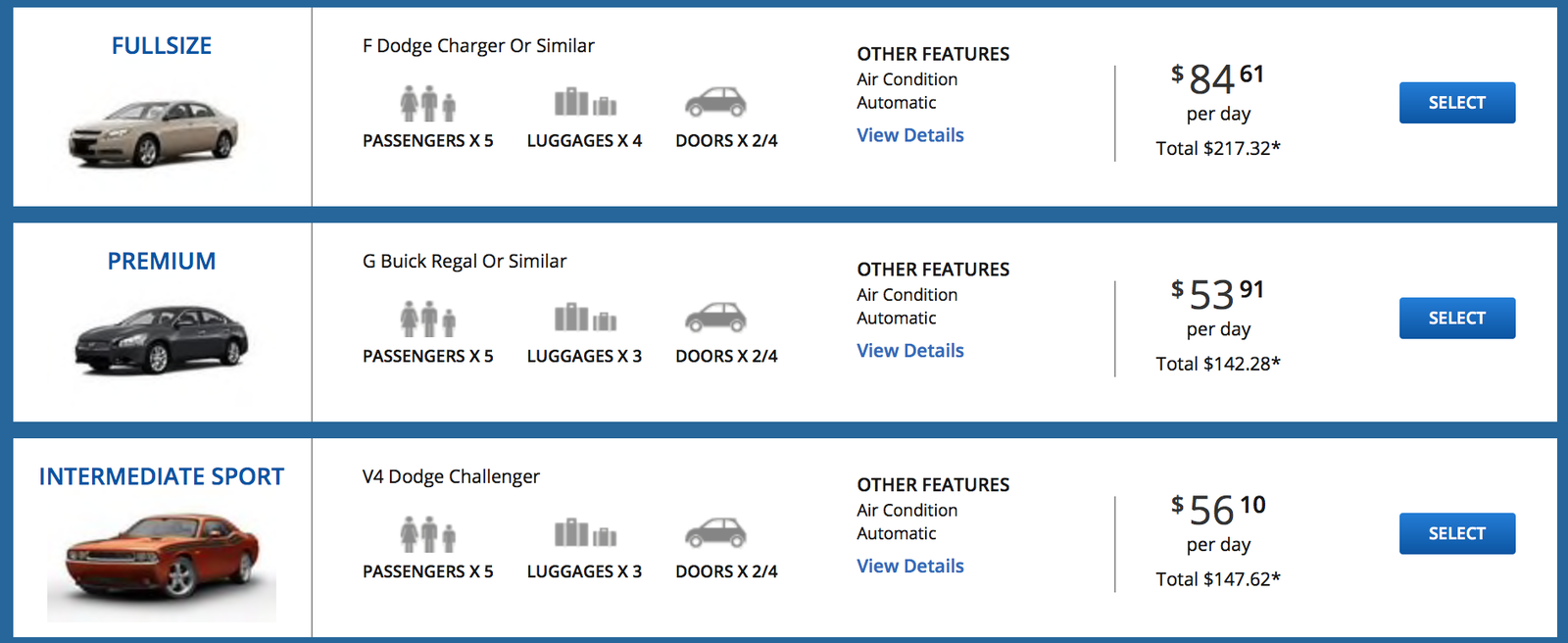The image is a screenshot from a car rental website, characterized by a prominent blue outline. Inside the blue boundary, the screenshot showcases three different car rental options. Each option features a distinct car type with respective details and pricing information.

1. **Full Size:**
    - **Car Model**: Dodge Charger or similar
    - **Visual**: The car is presented from a front-left angle, highlighting its left profile.
    - **Details**: Information includes the number of passengers, luggage capacity, number of doors, and other features. 
    - **Price**: $84.61 per day, with a total cost of $270.32 (marked with an asterisk).
    - **Action Button**: A blue "Select" button with white text underneath allows for selection.

2. **Premium:**
    - **Car Model**: Jeep, Buick Regal, or similar
    - **Visual**: The car is shown from a front-left angle, clearly displaying its left profile.
    - **Details**: Lists the number of passengers, luggage capacity, number of doors, and other features.
    - **Price**: $53.91 per day, with a total cost of $142.20 (marked with an asterisk).
    - **Action Button**: A blue "Select" button with white text underneath provides an option to choose this vehicle.

3. **Intermediate Sport:**
    - **Car Model**: Ford Dodge Challenger or similar
    - **Visual**: Depicted from a front-left angle, focusing on its left profile.
    - **Details**: Specifies the number of passengers, luggage capacity, number of doors, and other features.
    - **Price**: $56.10 per day, with a total cost of $147.62 (marked with an asterisk).
    - **Action Button**: A blue "Select" button with white text below it for selection.

Each car option prominently displays the "View Details" link in blue text, allowing users to access more comprehensive information about the vehicle features. The price is coupled with an asterisk, indicating the need for further clarification or conditions related to the costs.